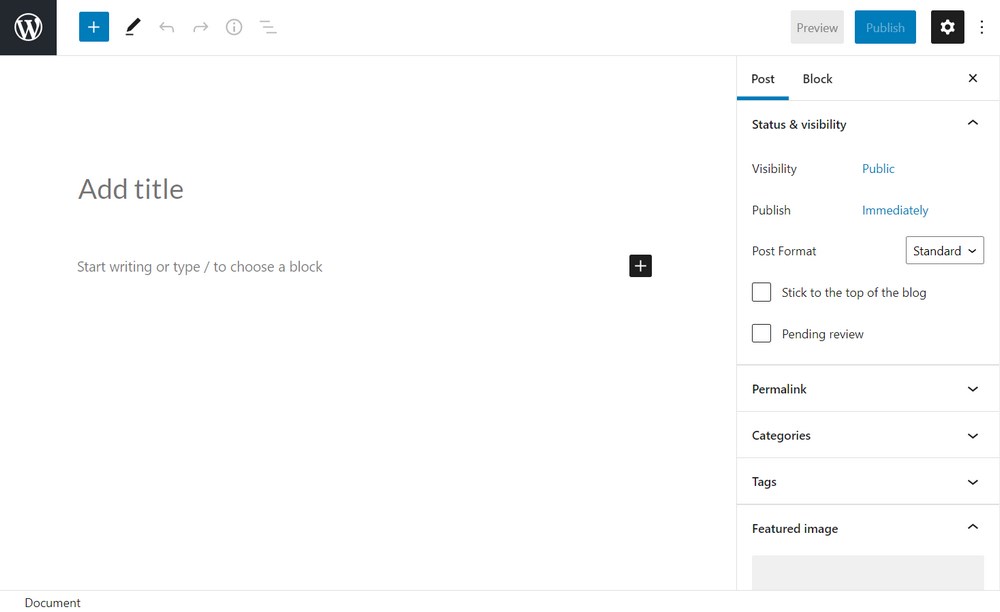The image showcases the WordPress website interface during the page-building process. In the top-left corner, a prominent WordPress logo is displayed: a white "W" inside a white circle, set against a black square background. Adjacent to it are several icons – a blue plus button, a black pen, and undo/redo options. Toward the upper-right side, there are additional navigation elements including "Help," "Preview," and a blue "Publish" button, accompanied by a white gear-shaped "Settings" icon set on a black background and a menu icon.

Centrally aligned to the left is a large white space designated for content entry. It prompts the user with "Head title" and "Start writing or type / to choose a block," with a black plus sign to the left indicating the option to add new blocks.

On the bottom left, there's a section labeled "Document." Towards the right, a pane reveals various post options. The "Post" tab is highlighted by a blue underline, displaying sub-options such as "Status and Visibility." Here, "Visibility" is set to "Public" and "Publish" is set to "Immediately," both highlighted in blue. The post format is marked as "Standard," and additional dropdown options for "Pending Review," "Permalink," "Categories," "Tags," and "Featured Image" are listed below.